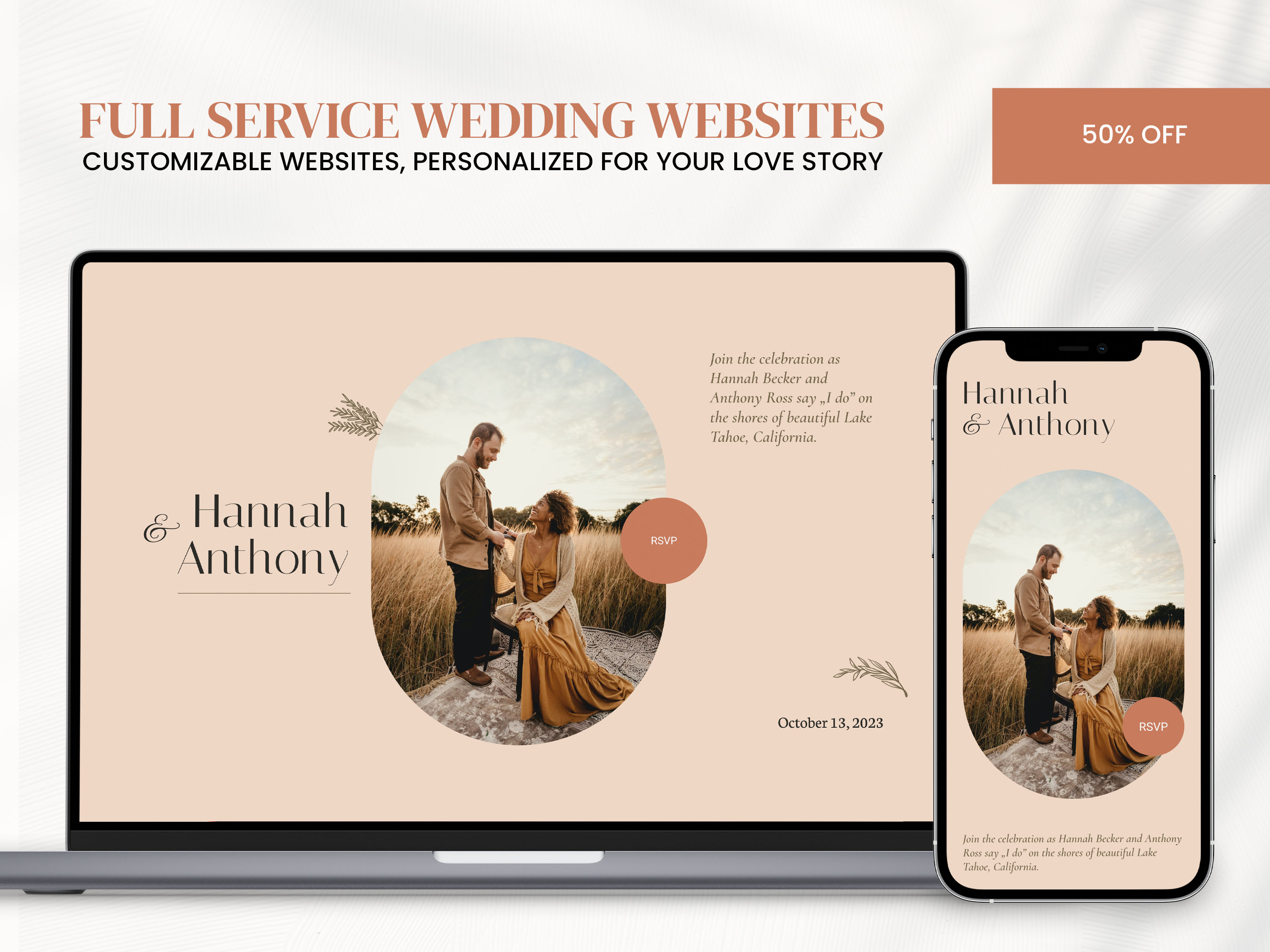The horizontally aligned rectangular image features a blended background of light gray and light brown hues. At the top, in medium brown all-caps text, the title reads "FULL SERVICE WEDDING WEBSITES." Below that, in smaller black all-caps text, it states "CUSTOMIZABLE WEBSITES, PERSONALIZED FOR YOUR LOVE STORY." To the right of this text, a small, brown-shaded rectangle announces "50% OFF" in white text.

The main section of the image showcases a computer screen and a cell phone placed side by side, both displaying a mock-up of a customizable wedding website. The screens feature a light tan background and prominently display the names "Hannah" and "Anthony." At the center of both screens is an oval-shaped photograph of the couple, Hannah Becker and Anthony Ross. They are outdoors, surrounded by tall brown grass, trees, and a sky with scattered clouds. In the photograph, Anthony is standing, looking down at Hannah, who is seated and gazing up at him.

To the right of the photograph on the large screen, the text reads: "Join the celebration as Hannah Becker and Anthony Ross say 'I do' on the shores of beautiful Lake Tahoe, California." Below this, on the lower right corner, the date "October 13, 2023" is displayed. The cell phone screen to the right mirrors this layout, presenting the same image and text. The overall aesthetic features a mix of reddish-brown, black, and cream colors, enhancing the natural and elegant visual theme.